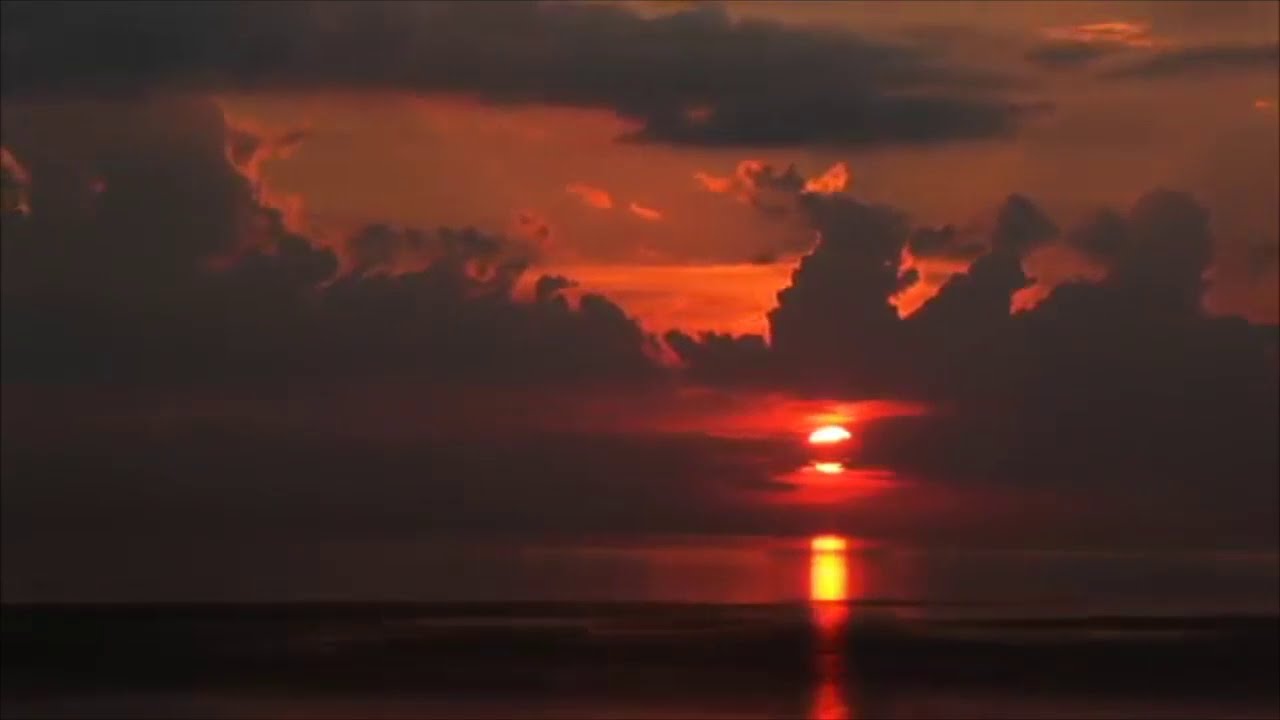The image depicts a dramatic sunset over a vast, tranquil body of water, either a calm ocean or a large lake. The sun, which is a bright white orb, is about two-thirds down the sky and two-thirds towards the right side of the photograph, still above the horizon. The image quality is slightly low resolution and details are subdued due to the intense lighting. Dark clouds partially obscure the sun, which casts a striking red hue onto the clouds immediately in front of it. These clouds stretch horizontally across the entire image and are primarily dark gray, while the clouds further in the distance glow with an orange tint, illuminated by the setting sun. Near the bottom of the image, a dark patch suggests the presence of shore or ground, but it's indistinct due to the dim lighting. Reflections of the sunset create a golden or red shimmering line on the calm, nearly motionless water below, adding to the serene yet vibrant atmosphere of the scene.